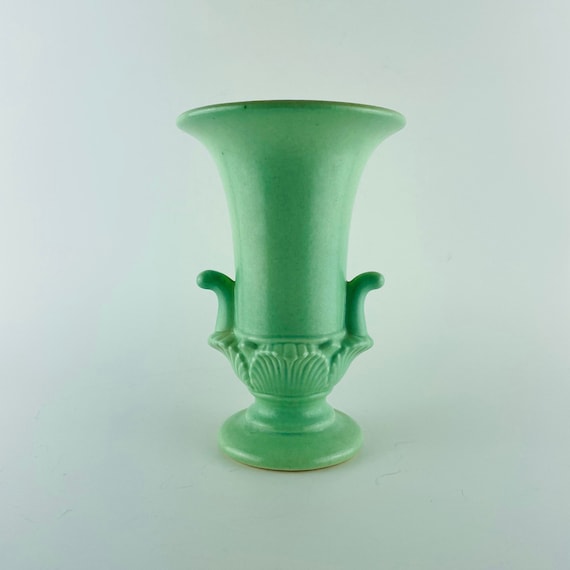This photograph showcases an antique-looking vase, possibly intended for display purposes such as an auction or sale. The square image features the vase set against an off-white to light gray background that seamlessly transitions into the white surface upon which the vase rests. The light green, almost salad-colored vase exhibits a combination of intricate and simple designs. 

At its rounded base, the vase rests on a small brown stand. Moving upwards, the vase narrows slightly before it fans out. The midsection of the vase features detailed leafy decorations on the front, left, and right sides, giving it an appearance of emerging from a flower. Near these decorations are two small, curved parts that resemble handles but are more decorative than functional. The vase then extends upwards into a long, tube-like neck, culminating in a large flared mouth at the top. Despite the fady and slightly foggy quality of the image, and its somewhat dark and grainy appearance, the vase's light green ceramic or clay material maintains a subtle shine.